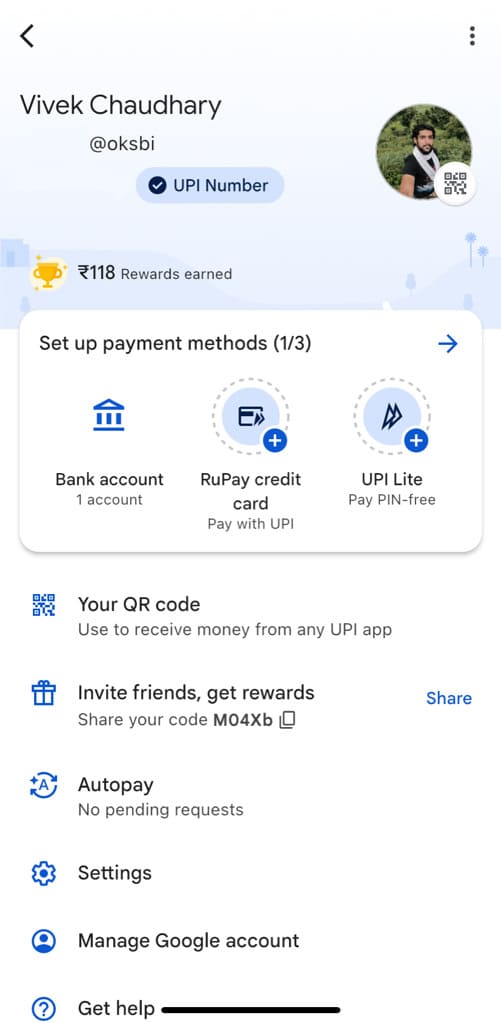Profile Summary of Vivek Chaudhary on Payment Platform:

The profile interface showcases the user, Vivek Chaudhary, with the username "OKSBI". The user interface includes a back arrow on the left and a vertical ellipsis (three dots) on the right for additional options. 

Highlighted Features:
1. **User Info**: Name displayed clearly as Vivek Chaudhary.
2. **Action Button**: A prominent blue button to view or change the UPI number.
3. **Rewards**: Indicates that Vivek has earned a total of 118 rewards.
4. **Setup Notification**: A pop-up setup guide is present, indicating “Set Up Payment Methods (1 of 3).”

Payment Methods Settings:
- **Bank Account**: One account already set up.
- **RuPay Credit Card** and **UPI Lite**: Options available with a "+" icon indicating they have not been added yet.
- **Payment Configuration**: There is an option to enable PIN-free payments with UPI Lite.

Additional Features:
- **QR Code**: Displayed "Your QR code used to receive money from any UPI app."
- **Referral Program**: Option to "Invite Friends, Get Rewards" with an opportunity to share a referral code: MOXMO4XB.

Background:
- Light blue background providing a clean and user-friendly interface.

This detailed layout of the profile offers a comprehensive overview of the user's interface, payment setup progress, and additional interactive options.